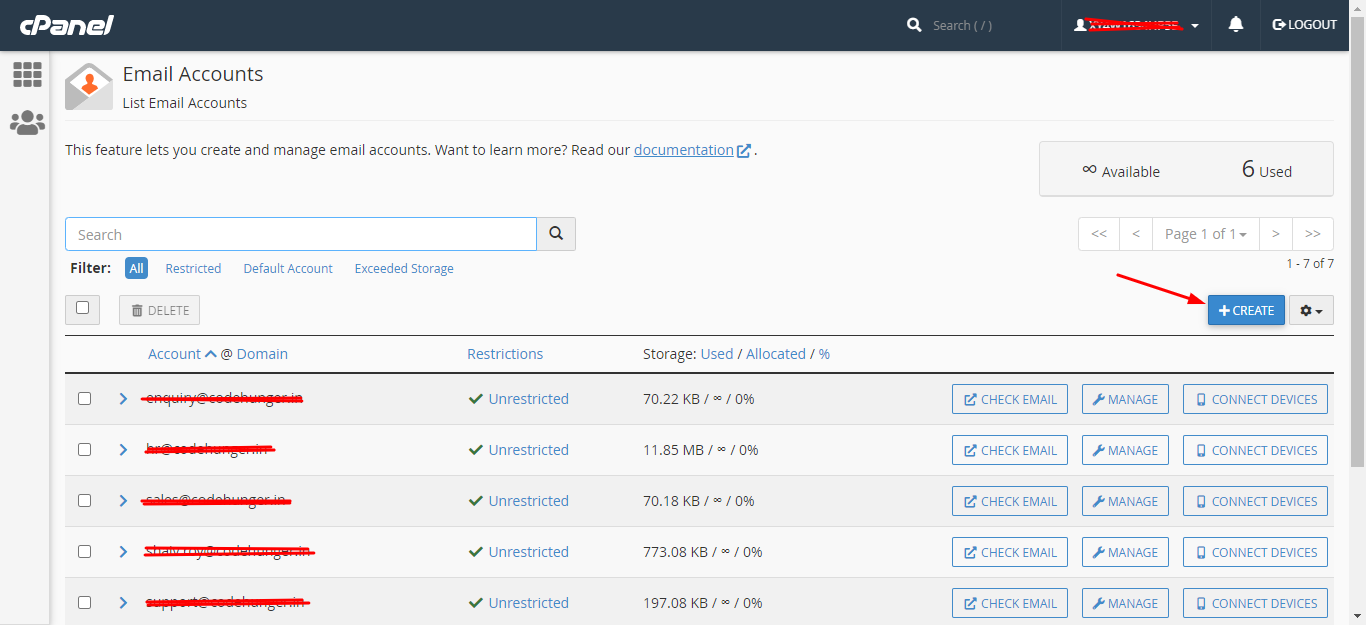The image displays the user interface of an application within its cPanel. The cPanel features a dark background at the top, integrating a search box. Key options such as notifications and logout are displayed, with the username appropriately hidden for privacy. The interface prominently presents the section titled "Email Accounts," with a subheading "List Email Accounts." A description follows, explaining that this feature allows for the creation and management of email accounts. A prompt to "Read our documentation" is also included, with the word "documentation" highlighted in blue.

Below this, there is another search bar and an "All" filter. The interface lists email accounts and their associated domains, with all email addresses obscured by red lines to protect personal information. The email list is organized into three columns. The first column indicates the account and domain. The second column shows restriction statuses, all marked as "Unrestricted" accompanied by a green tick. The third column details the storage usage, with the following values listed: 70.22 KB, 11.8 MB, 7.18 KB, 773.08 KB, and 197.08 KB.

Additionally, each row features functional buttons labeled "Check Email," "Manage," and "Connect Devices," all presented in blue squares. On the right side of the interface, there is an indicator showing "6 Used" and "Available," and a "Create" button for adding new email accounts, highlighted by a red arrow pointing towards it.